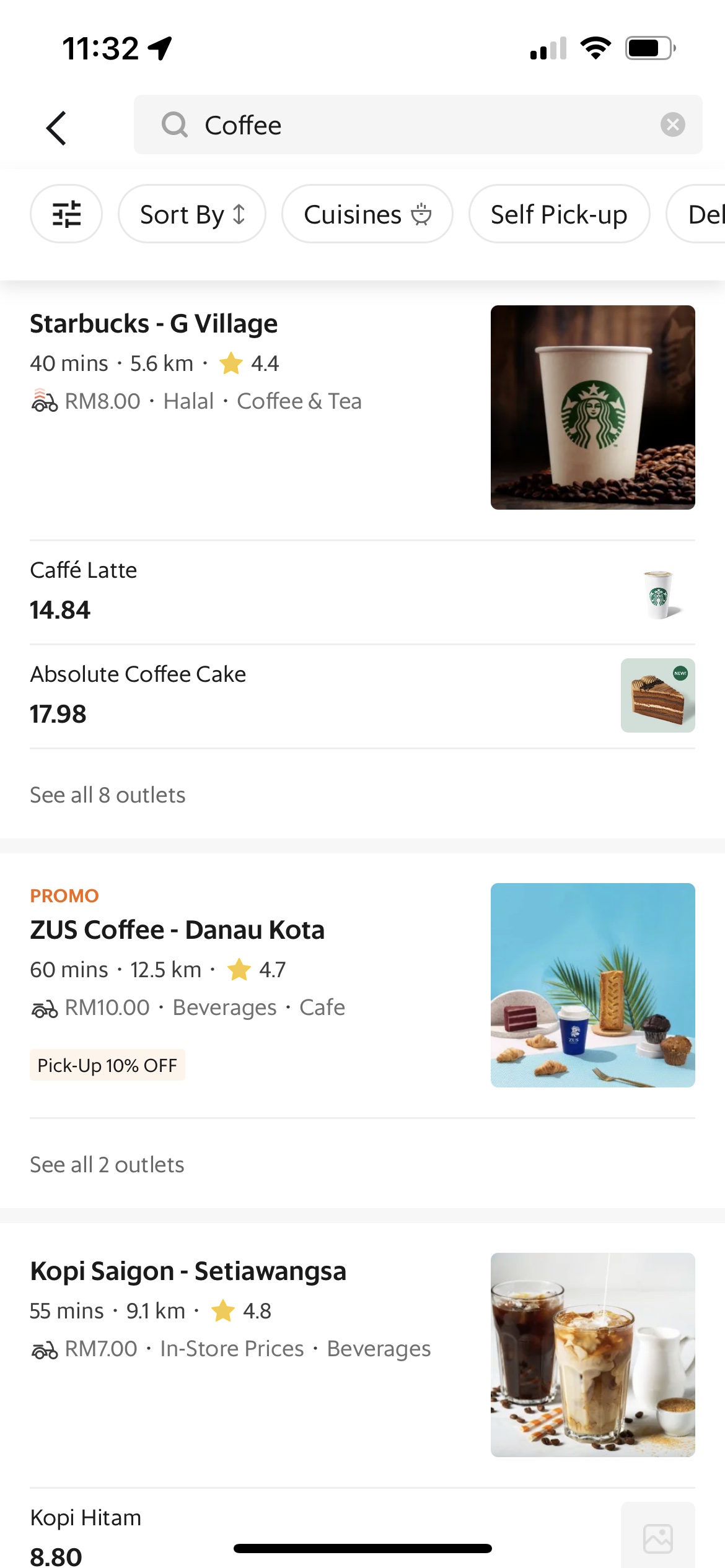The vertically-oriented, rectangular image appears to be a screenshot taken from a smartphone, capturing someone’s search for coffee. At the very top left corner, the current time is displayed as 11:32 in black text. On the top right, there are indicators for signal strength showing two bars, Wi-Fi strength at full, and a battery icon approximately three-quarters full.

Below these indicators, a gray search bar displays the word "coffee" in black text. Directly beneath this search field, options for sorting search results are partially visible, including "Sort by," "Cuisines," and "Self-pickup," with additional options being cut off by the bottom edge of the image.

The first search result prominently features "Starbucks G Village" in bold lettering, accompanied by details such as an estimated 40-minute bike ride to the location, a cost of RM8.00, and a description noting its offerings of halal coffee and tea. There is a small image of a Starbucks coffee cup adjacent to this information. The next entry within the same section includes "Cafe Latte" and "Absolute Coffee Cake," suggesting various menu options available at this Starbucks location. Additionally, there is a link stating "See all eight outlets in this section."

Below this, a promotional listing for "Zeus Coffee" is displayed. The details mention delivery in 60 minutes, a price of RM10.00, and highlight available beverages and café items, alongside a 10% pickup discount. An image featuring coffee and other items accompanies this promotional entry.